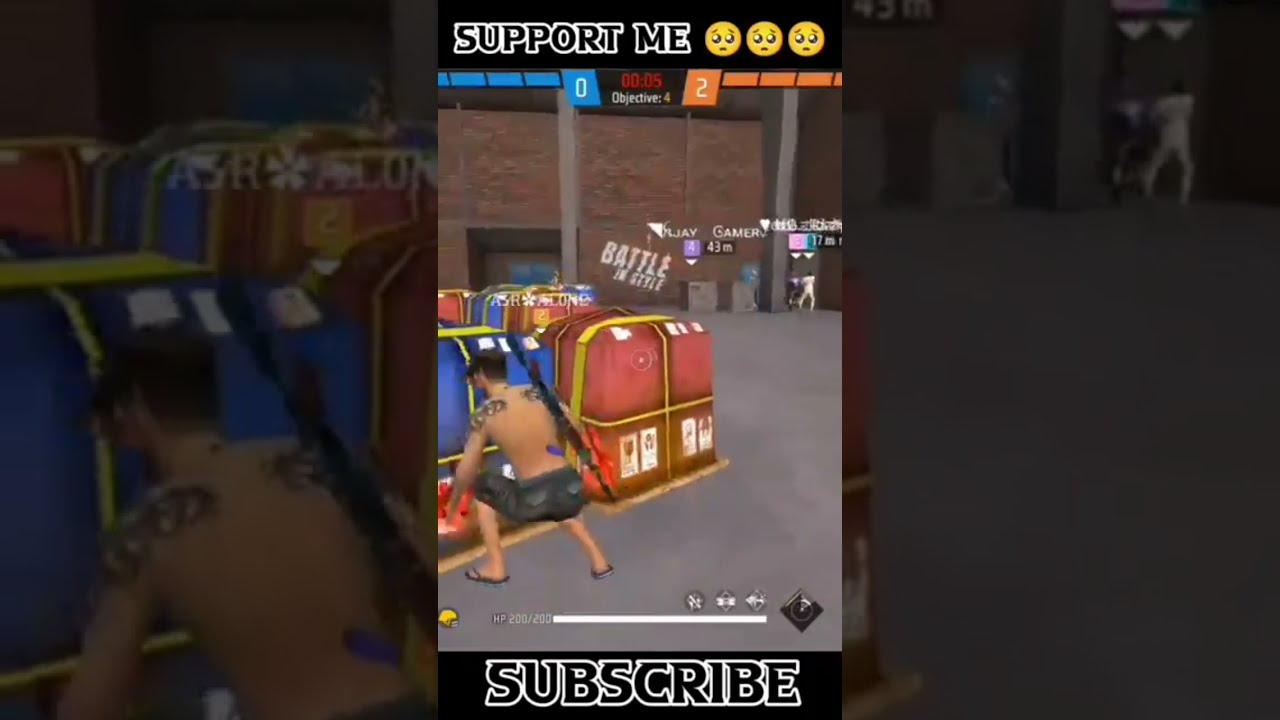The screenshot is from a slightly cartoonish video game, capturing a shirtless animated figure with dark hair and light brown skin. The figure, adorned with black tattoos over both shoulders and wearing black pants and sandals, is kneeling down with a gun strapped to their back. Positioned in front of the character are two large, ornate crates: one blue with yellow designs and the other red with gold designs. More similar crates are visible in the background, partially obscured. The setting appears to be a warehouse or a large open building featuring gray flooring and a distant brown brick wall with the text "Battle and Style" on it. Above the character, white text on a black background reads "support me" accompanied by three sad-faced emojis. A digital time clock with red writing is centered below this, flanked by score indicators showing 0 for the blue team and 2 for the orange team. At the bottom of the image, the words "subscribe" appear in white font against a black background. The screenshot sits prominently in the middle third of the entire image, with the left and right portions showcasing zoomed-in, darkened versions of the central image.